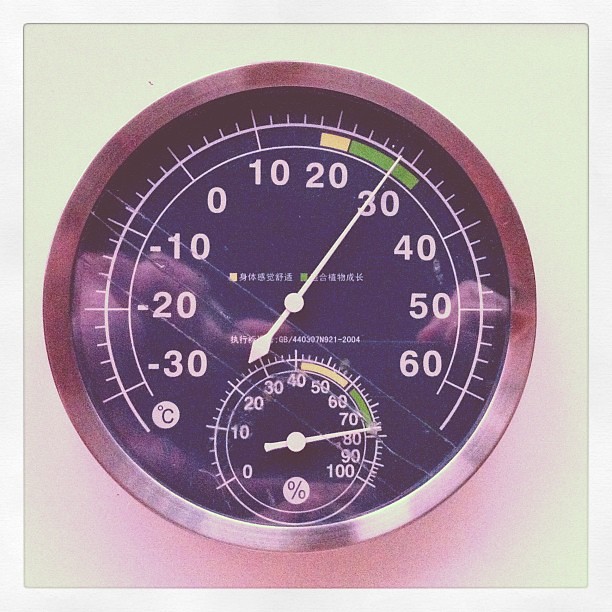This image features a detailed close-up of a thermometer and hygrometer placed on a white surface. The device, encased in a silver frame, combines both temperature and humidity measuring instruments in one dial. The larger, outer circle of the dial is designated for temperature measurement, marked in both Celsius and Fahrenheit. The scale ranges from -30°C to 60°C, with a green bar highlighting the optimal temperature range between 20.2°C and 30.2°C. Currently, the temperature pointer indicates approximately 30°C. 

Positioned at the lower center of the main dial, a smaller circle displays humidity levels, scaled from 0% to 100%. The humidity indicator shows 80%, which falls within the upper limit of the optimal humidity range, highlighted in yellow from 40% to 60% and green from 60% to 80%. 

The overall tone of the photo is subtly yellowish, adding a warm hue to the image. The black background of the device's face contrasts sharply with the white numerical and scale markings, enhancing readability and emphasizing the instrument’s functionality.